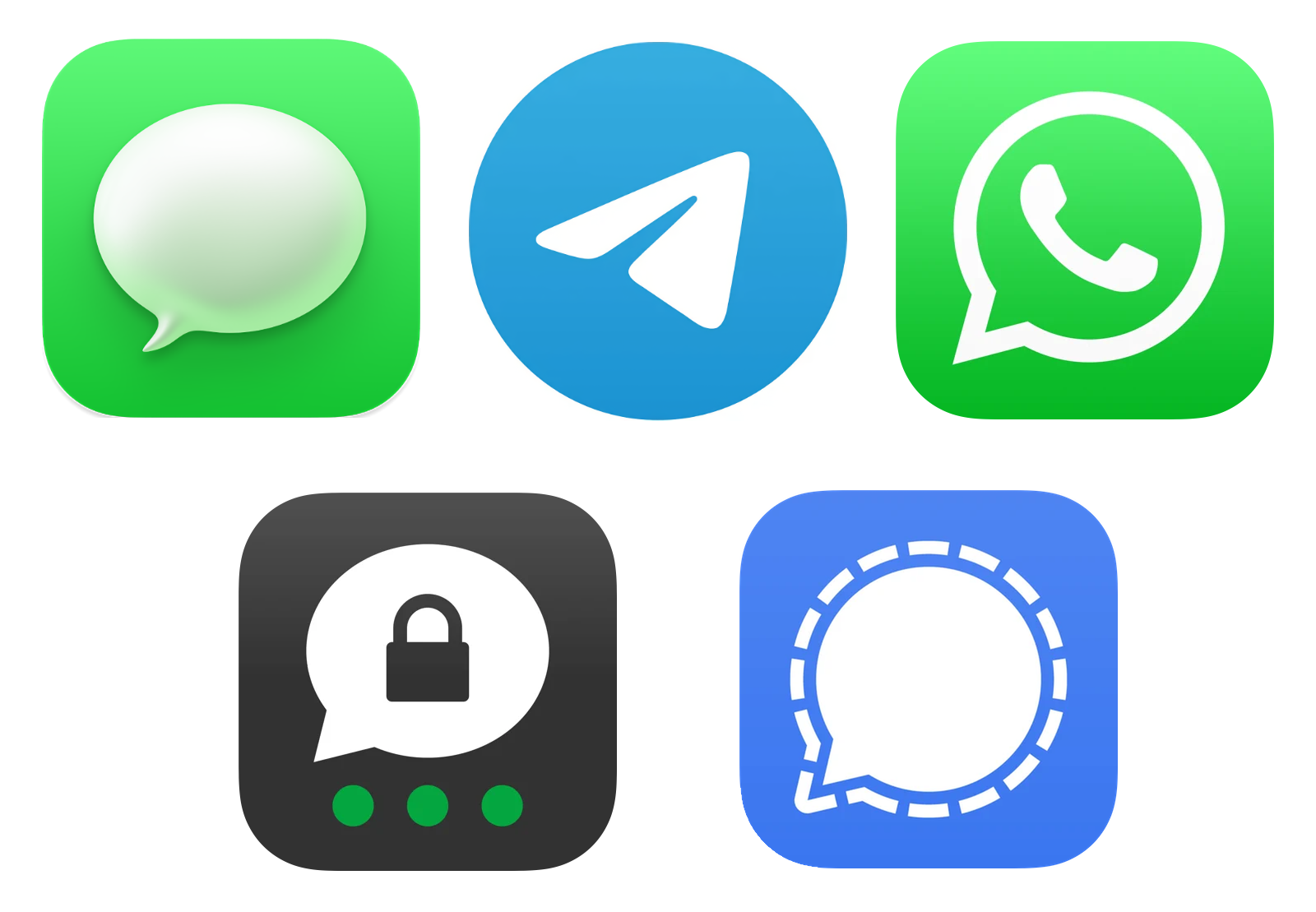The image displays five app icons arranged in two rows on a phone, with three icons in the top row and two in the bottom row, all featuring rounded corners indicative of iPhone apps. The top left icon is a green square with a white speech bubble, reminiscent of the Messages app. To its right is a dark blue circular icon with a white triangle, which could represent the Telegram app. The top right icon is another green square, but with a white speech bubble containing a telephone receiver, similar to the WhatsApp icon. On the bottom row's left side, there is a black square with a white speech bubble enclosing a black lock and three green dots below, possibly indicating a security or passcode app. The final icon on the bottom right is a blue square featuring a white speech bubble, which has dashed lines surrounding it, suggesting it might be related to messaging or communication.